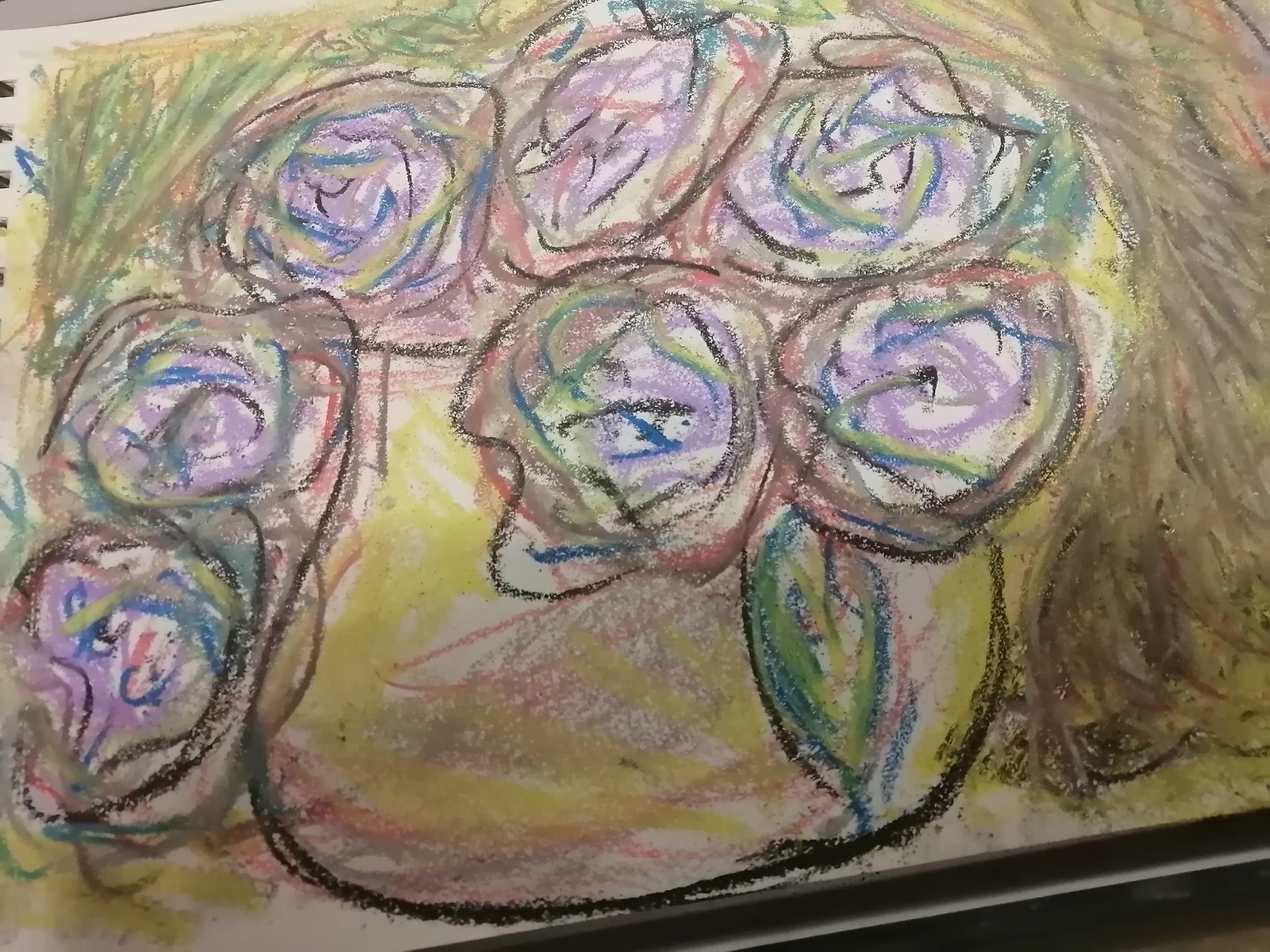The photo captures a drawing from an open sketchbook, with a faint view of the edge and spiral binding in the top left corner. The drawing, primarily done in pastels and colored pencils, depicts a vase filled with a bouquet of seven rounded, crudely drawn flowers and a single visible leaf. The flowers, appearing somewhat like roses, display interior swirls and depth. The vase itself is shaded with yellow, while the blooms exhibit hues of blue, purple, pink, and hints of brown and green. The background is filled with thick, earthy tones of brown and green crayon strokes, reminiscent of a simple still-life setting. The image is devoid of text, people, animals, buildings, or mechanical objects, leaving the focus solely on the childlike, yet timeless, floral illustration.